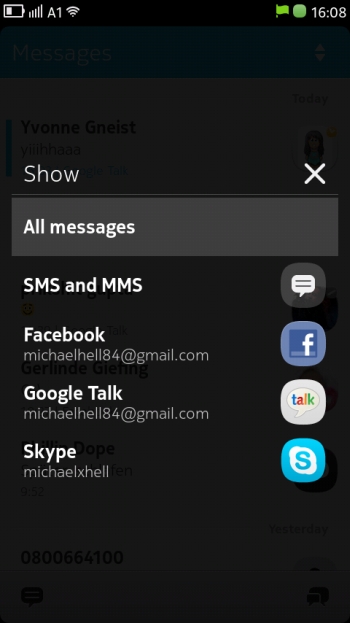The screenshot, taken from an older Android smartphone, reveals a cluttered interface indicative of multiple communication apps in use. In the top-left corner, the status bar displays an almost empty battery icon, full signal strength, "A1" as the carrier, and a full Wi-Fi signal. On the top-right, a flag icon in a whitish or greenish-yellow hue is shown, followed by a green circular icon with "1806" in white text. The screen then fades into a dark, black space.

Beneath this, there is a "Show" button on the left and an "X" on the right, flanking a grayish box with the text "All Messages" in white. Below this box, a white string of letters "MSMSMSMMS" appears. To the right, a gray circle encloses a white speech bubble icon.

Further down is a section titled "Facebook" in white text, accompanied by the user's email address in gray. On the far right of this line, the Facebook logo is displayed in blue and white. Following that, the next line reads "Google Talk" alongside the user’s email address in gray, with the now-discontinued Google Talk logo on the right.

At the bottom of the screenshot, "Skype" is listed with the user's Skype name in gray, paired with the familiar white and blue Skype logo on the left. This collection of details points to a dated interface, reflective of a time when these communication platforms were widely used.